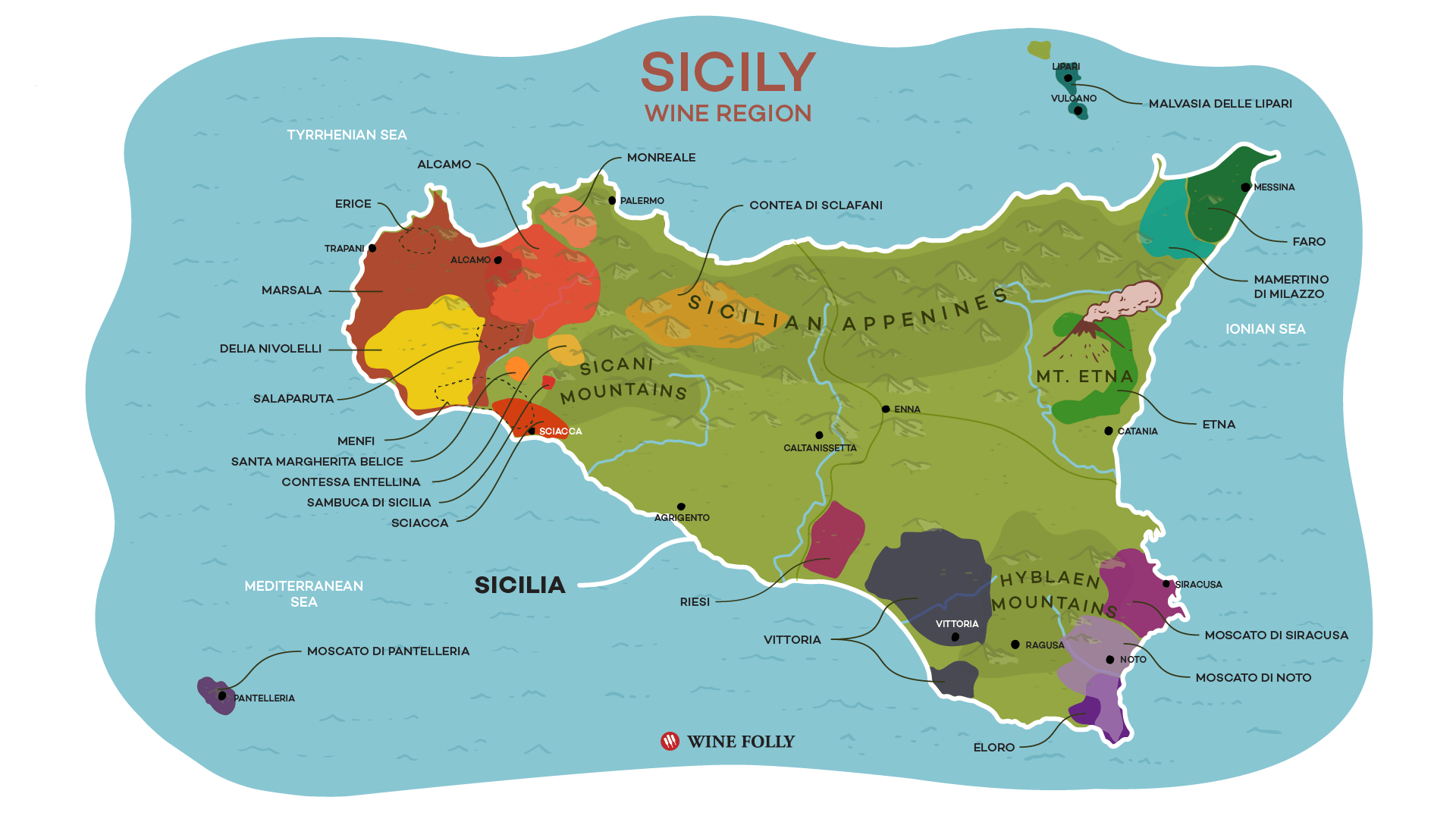This illustrated map prominently features the "Sicily Wine Region" title in striking red at the very top center. Surrounding the landmass is a light bluish-green background, evoking the sea with subtle, darker blue wave illustrations. The map's border is curvy and wavy, enhancing its aesthetic appeal.

Dominating the center is the landmass of Sicily, depicted in varied hues. The core of the island is primarily light and dark green, punctuated by regions with distinct colors. To the far top left, the areas are colored in browns, yellows, reds, and oranges. The very top right showcases darker greens transitioning into teal, and you can see Messina and Pharaoh labeled in black text. Central right is an artistic depiction of Mount Etna, clearly labeled in black. The lower right portion of the island is shaded in purples, both dark and lilac, with smatterings of gray.

Additionally, various areas across the landmass are marked with text denoting key wine regions and points of interest, such as the Sicilian Alpines at the top with an adjoining orange patch identified as Cantia de Sclafani or Sclafen. Three seas marking the surrounding waters—Tyrrhenian Sea at the top left, Mediterranean Sea at the bottom left, and Ionian Sea on the right edge.

At the bottom left as well as the top right, small islands can be observed. Anchoring the map at the very bottom center is the text "Wine Folly" in black, accompanied by a small red logo, emphasizing the thematic focus of the map on the Sicilian wine territories.